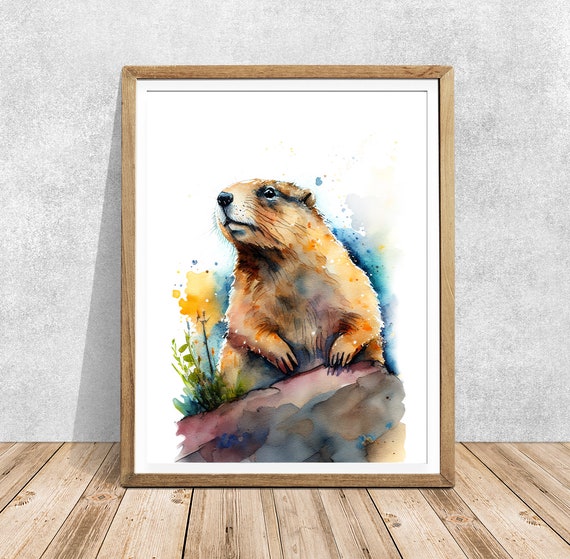This image displays a framed watercolor painting of an otter, presented in a medium, unfinished wood frame. The frame rests against a gray wall on a wooden floor. In the painting, the otter is centrally positioned, surrounded by a white background. The artwork features a palette of brown, yellow, blue, and purple tones. The otter, rendered in varying shades of dark and light brown, gazes contentedly toward the viewer's left. He sits atop a large, reddish-brown rock, which dominates the lower portion of the painting. To the otter's left, there are yellow flowers and a couple of grass sprouts, adding a touch of nature to the composition. The overall style is slightly abstract, appealing to animal lovers and fitting for display in a living room or office.